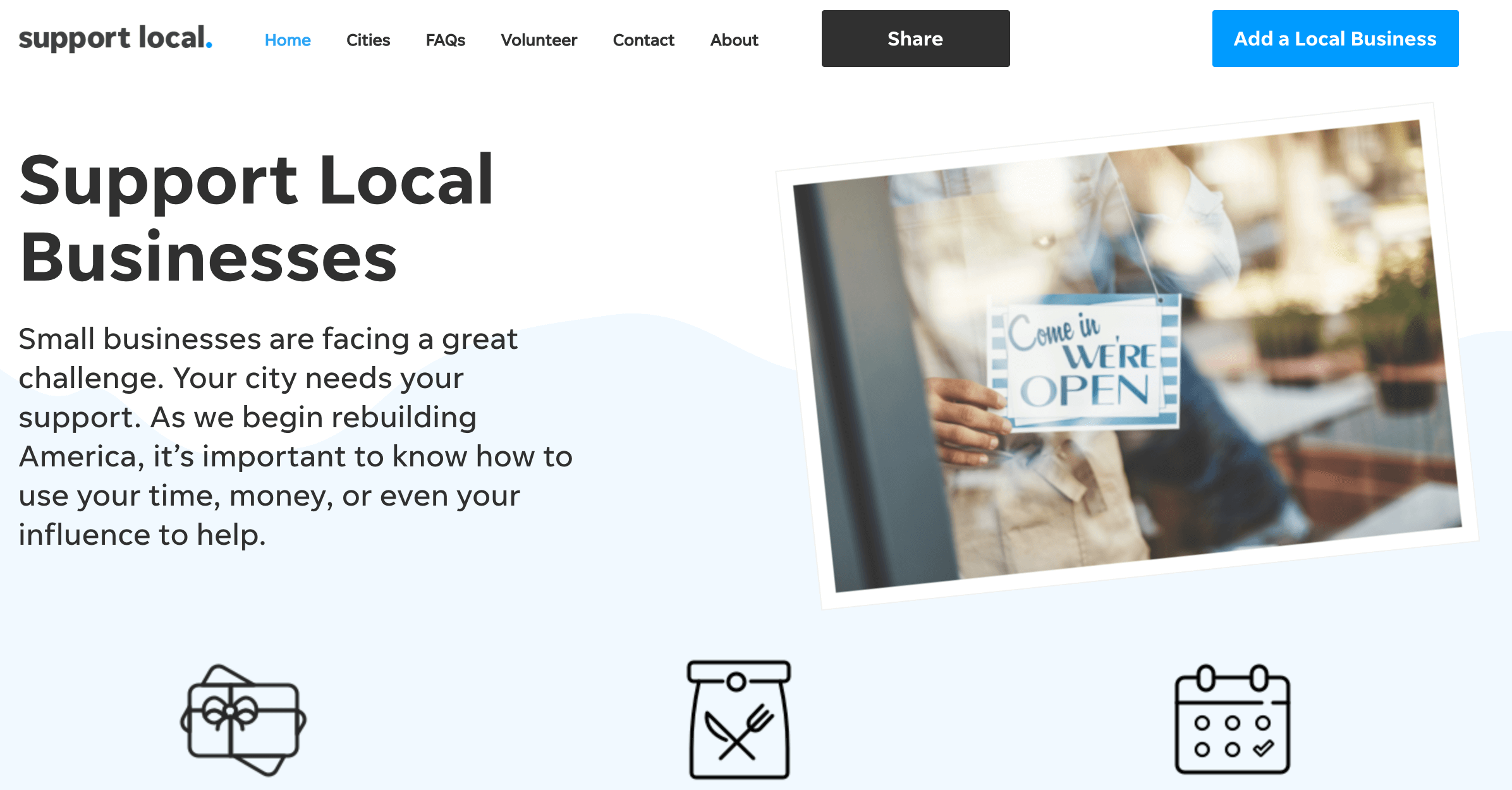The top left corner of the image features a black text reading "Support Local" followed by "Homes" in blue, possibly indicating the current section or location within the site. Various navigation tabs are present, including "Cities," "FAQs," "Volunteer," "Contact," and "About." 

There is a black rectangle with white text labeled "Share," and next to it, a blue rectangle with white text that reads "Add a Local Business." Below these, a heading in black states, "Support Local Businesses." The accompanying paragraph describes the challenges local businesses are facing: "Local businesses are facing a great challenge. Your city needs your support. As we begin rebuilding America, it's important to know how to use your time, money, or even your influence to help."

The image showcases a person inside a window holding a blue and white sign that says, "Come in, we're open," indicating an operational business.

At the bottom left of the image, there are three icons against a light blue background:
- The first icon is a black outline of a rectangular gift with a ribbon.
- The second icon depicts a bag containing a fork and knife, also in black outline.
- The third icon resembles a calendar or organizer with two notches at the top. It features five circles arranged with three on top and two below. The circle on the bottom right is checked.

This image and its elements focus on encouraging support for local businesses amidst their ongoing challenges.